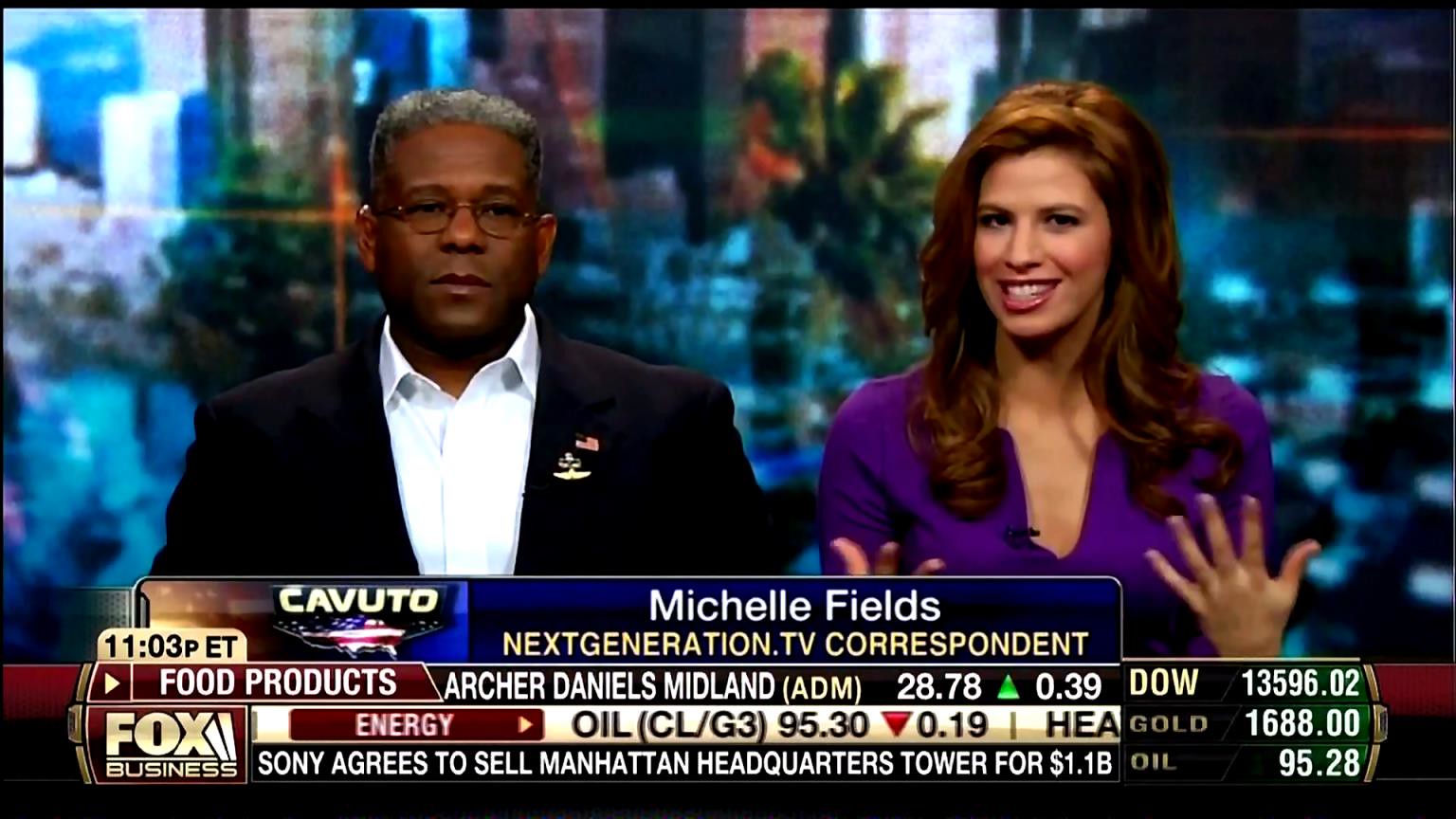This detailed still shot captures a Fox Business television broadcast featuring two newsreaders in front of a blurry backdrop depicting a cityscape with buildings, lights, and plants. On the left, an older man with black and silver hair, who is wearing wire-framed glasses, a blue blazer adorned with a flag pin and another badge, and a white shirt, faces the camera. To his right, a younger woman named Michelle Fields, identified as the "Next-Generation TV Correspondent," is smiling and gesturing with her hands. She has short, shoulder-length reddish-brown hair and is dressed in a purple blouse. Below them, multiple lines of text provide various details such as the time "11:03 PM ET" and a stock ticker that includes "Food products Archer Daniels Midland (ADM) 28.78 ▲ 0.39," "DOW 13596.02," "Oil (CL-G3) 95.30 ▼ 0.19," and "Gold 1688.00." The bottom line of the ticker reads "Sony agrees to sell Manhattan headquarters tower for $1.1 billion." The Fox Business logo is prominently displayed in the bottom left corner of the screen.